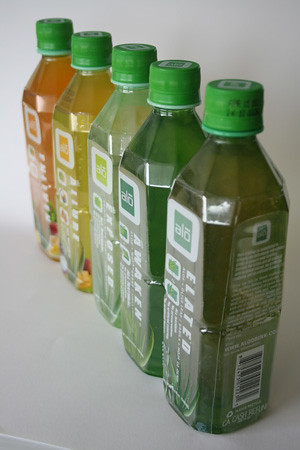In this image, there are five bottles of a beverage, likely juice, arranged diagonally from the upper left to the lower right corner. The bottles, all of equal volume, display a gradient of colors, starting with orange on the upper left, followed by yellow, light green, dark green, and ending with the darkest green on the lower right. Each bottle's label, although partially obscured, is visible enough to discern the brand name "Aloe" (A-L-O). The labels also indicate different purposes: the bottle closest to the viewer is labeled "elated," and the one next to it reads "awaken." The exact purposes of the other beverages are hard to read due to their less visible labels.